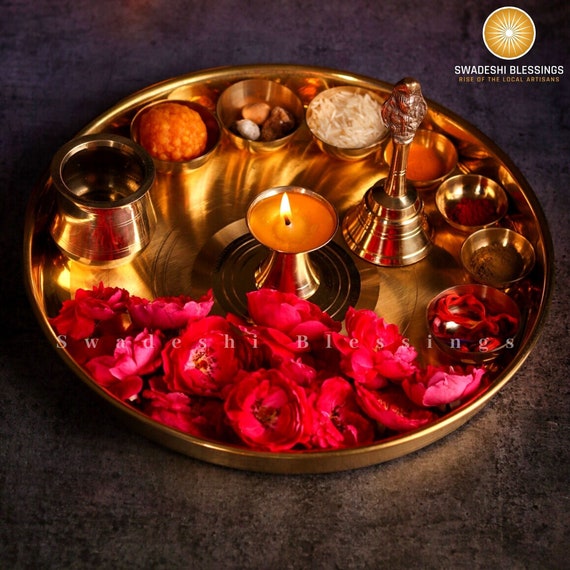This image showcases a beautifully arranged gold circular tray adorned with various floral pieces and offerings. The centerpiece of the tray is a lit candle in a brass-colored holder with a vivid yellow flame. Surrounding the candle are an array of small metallic bowls, each holding different items including nuts, rice, spices like turmeric, cumin, and paprika, as well as chickpea chutney, dried dates, and potentially cut-up coconut. There are also bowls containing a muffin, potpourri, and red roses. A small brass dinner bell with an engraved handle is positioned to the right of the candle. The tray itself is shallow and polished, capturing the warm glow of the candlelight. The image is titled "Swadeshi Blessings," hinting at a celebration of local artisans, with the offerings and symbols reflecting a rich cultural tradition.